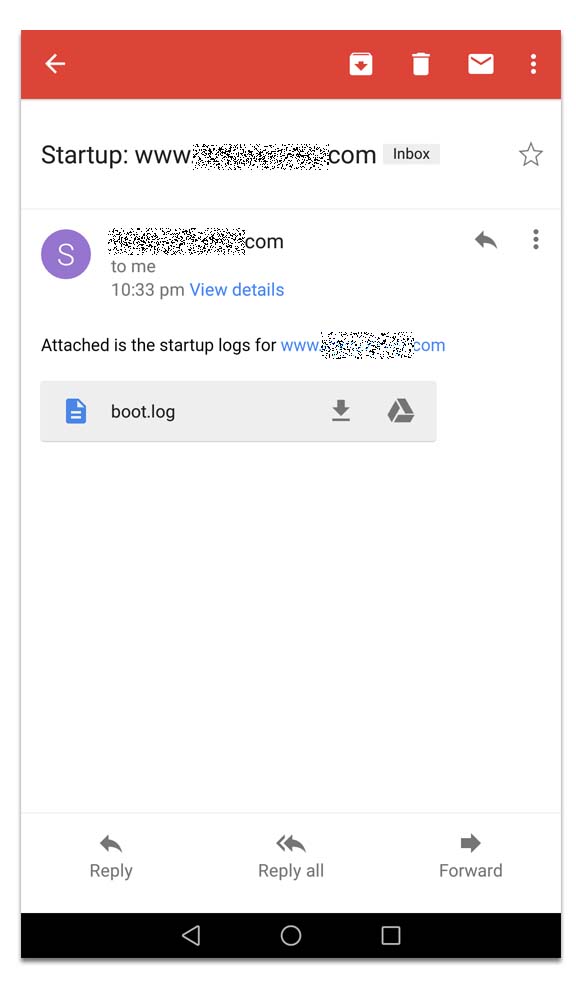This is a detailed caption for the image:

The screenshot appears to have been taken within a mobile app on a phone. At the very top of the screen, there is a red bar. On the upper left-hand side of this bar, there is a left-pointing white arrow. Moving towards the right from the center of the red bar, there is a white rectangular box with a red downward-pointing arrow to its left. To the right of this box, there is a white trash can icon, followed by a white envelope icon. Next to the envelope, there are three vertically aligned white dots.

Just below the red bar, the text "startup www[blanked out]com inbox" is displayed. Beneath this text, there is an icon that appears as a letter "S." To the right of this icon, there is a blanked-out area followed by the text "com." Below this, the phrase "to me" is shown, and directly underneath it, the time "10:33 p.m." is displayed. To the right of this timestamp, the words "view details" in blue font can be seen, accompanied by a forward arrow icon and three vertical dots.

Continuing down the screen, on the left-hand side, there is a message that says, "Attached are the startup logs for www[blanked out]com." Below this message, a link to "boot.log" is presented, offering options to download the file or to send it to Google Drive. At the bottom of the screen, there are options available to "Reply," "Reply All," or "Forward" the email.

This screenshot captures the interface of an email within a mobile app, showing various options for managing and interacting with the email and its attachments.